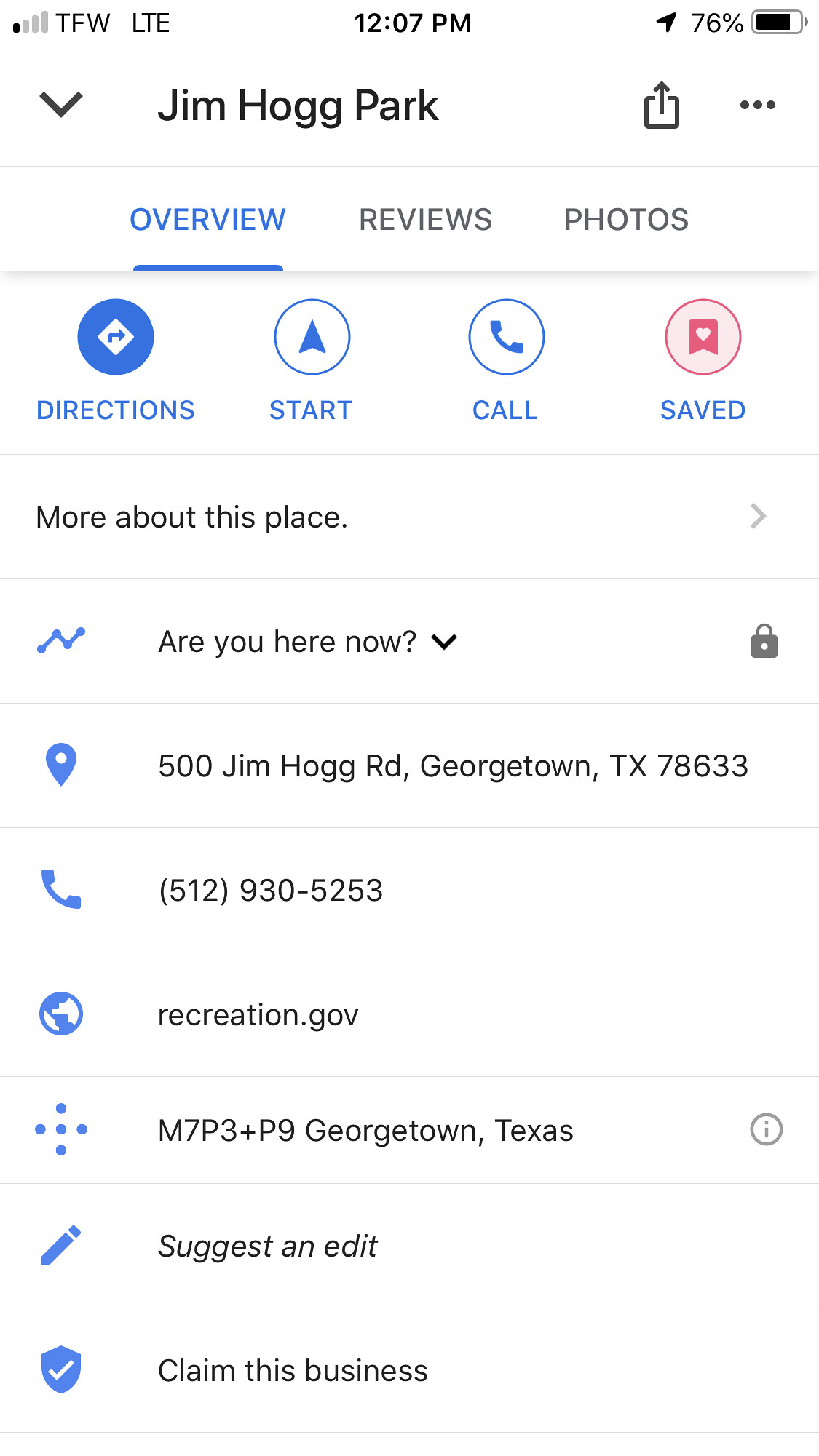The image depicts a screen from a mobile app showcasing details about Jim Hogg Park. At the very top of the screen, various mobile phone icons are displayed. Directly below, the title "Jim Hogg Park" is prominently featured. Underneath the title, three tabs are displayed: "Overview" (highlighted in blue and currently selected), "Reviews," and "Photos."

Below the tabs, four interactive options are arranged in a row:
1. **Directions:** Indicated by an arrow pointing to the right.
2. **Start:** Indicated by an arrow pointing upwards.
3. **Call:** Represented by a phone call icon.
4. **Saved:** Depicted with a bookmark icon containing a heart.

Following these options, the text "More About This Place" is found, accompanied by a gray arrow pointing to the right. The subsequent row asks, "Are You Here Now?" with a lock symbol adjacent to it.

The following information is provided:
- Address: 500 Jim Hogg Road, Georgetown, Texas, 78633
- Phone number: (512) 930-5253
- Website: Recreation.gov
- Plus Code: M7P3+P9, Georgetown, Texas, with a gray information symbol next to it.

Finally, two additional interactive options appear at the bottom:
- "Suggest an Edit"
- "Claim This Business"

All rows and sections are neatly separated by thin light gray lines, ensuring a structured and organized presentation.